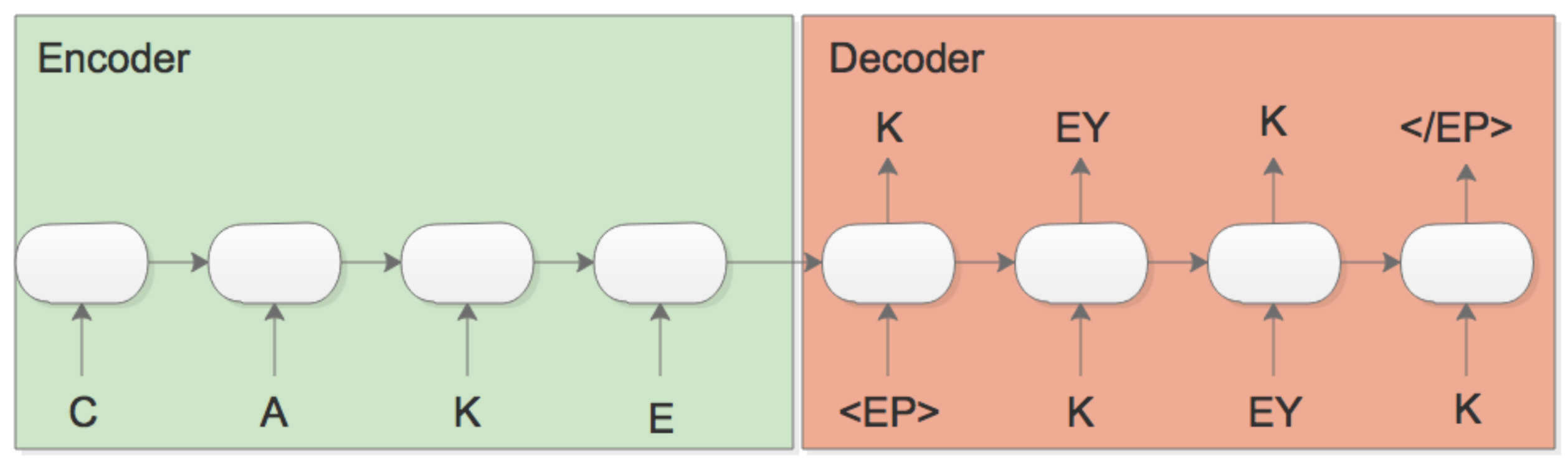This detailed image features an encoder and a decoder, likely illustrating a basic cryptographic process. On the left side, the encoder section has a green background with four white buttons marked with the black letters 'C', 'A', 'K', and 'E'. Arrows connect each button to the next, leading towards the right. The adjacent decoder section has an orange-brown background and is similarly structured with white buttons containing the black letters 'K', 'EY', 'K', and a symbol that appears as '(E/P)'. Below these primary buttons in the decoder are additional buttons labeled 'E-P', 'K', 'E-Y', and 'K', each aligned with arrows pointing upwards to their corresponding top button. The image lacks accompanying text to explain its purpose, but it seems designed to visually represent the basic function of encoding and decoding information.